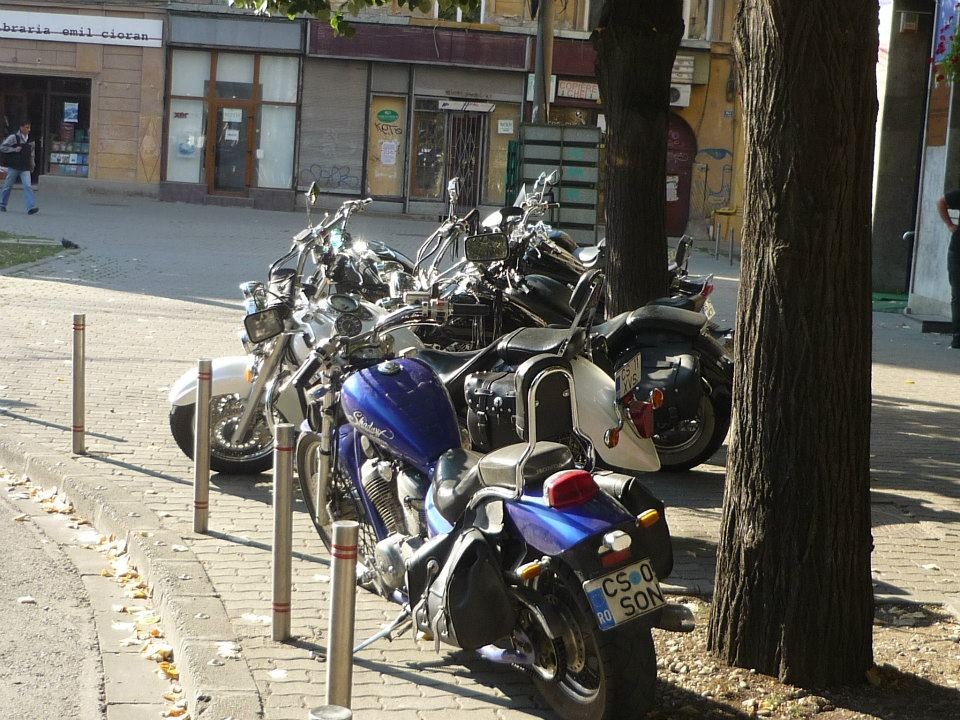This detailed color photograph captures an urban scene centered around three motorbikes parked on a brick-paved sidewalk with a wavy pattern. The foreground prominently features a blue motorcycle with a white "Shadow" decal on its fuel tank and a license plate that reads "CS0 SON" beneath a red taillight. Adjacent to the blue bike, a couple of motorbikes in white and silver hues are arranged in a line. Beyond the pavement's edge in the bottom left corner, a curved roadway is visible, bordered by four short metal poles adorned with red stripes at the top and bottom. Scattered white and yellow petals lie near the curb. The right side of the image shows a large, dark tree trunk close to the blue motorbike, and another tree further back toward the center. In the upper left-hand corner, a person in a grey and black jacket and jeans, carrying a black bag, is walking towards the center of the image, near a small triangular patch of grass on the sidewalk. The background reveals a series of grey and beige commercial buildings with maroon and white signs, although the text on these signs is not readable.